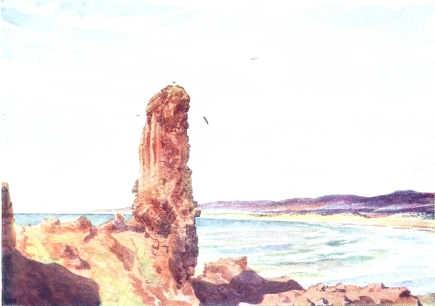The painting portrays a dramatic coastal scene dominated by a towering rock formation that juts out from the side of a cliff near a serene sea or bay. The colossal rock, much like a giant cucumber or an ancient totem, appears naturally shaped by the elements and stands prominently in the foreground. It is composed of a palette of browns, yellows, and subtle oranges, exuding an almost pinkish coral hue. A shadow cast by the sun accentuates the texture and height of this imposing structure, which faces a light blue, green-tinted expanse of water. Below and around this main rock, a series of rocky outcroppings deepen the complexity of the landscape. Further back, beyond the gentle waves, a stretch of sandy beach or light brown-yellow shoreline meets the horizon, which is beautifully framed by low, purplish foothills. The sky above is predominantly white with just a hint of blue, adding a serene, almost ethereal quality to the scene. An almost imperceptible bird might be seen flying near the towering rock, adding a touch of life to this tranquil, almost otherworldly coastal vista.